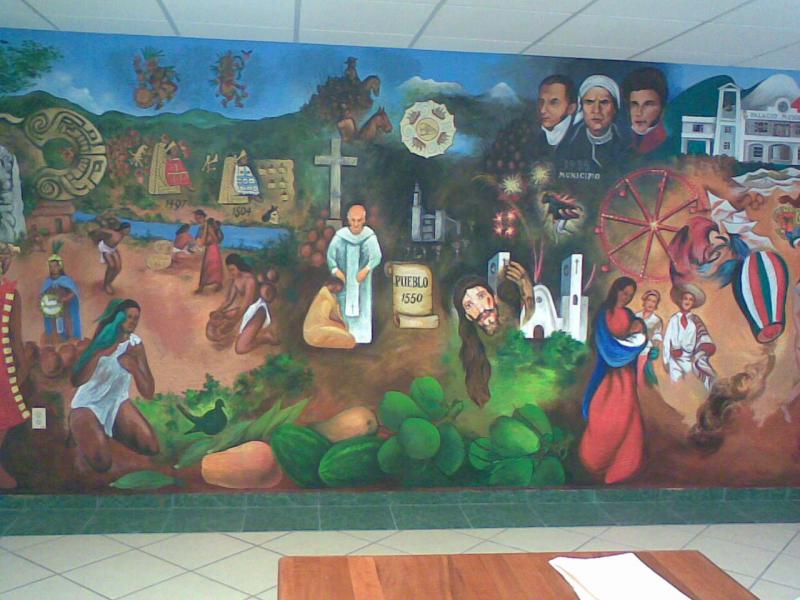This image captures a large, detailed mural that prominently showcases Christian themes and historical elements, likely representing Mexico's rich Christian history. The mural, set against a white background, includes a variety of vivid colors such as green, brown, red, white, aqua, dark green, and royal blue. At the center, there's a depiction of Jesus carrying the cross, with only his head and part of the cross visible. Around him, various other figures and activities are portrayed, including a priest placing his hand on the head of a kneeling native figure dressed in light orange.

To the right of this central scene, numerous European figures are depicted, alongside a modern plantation-style house at the top right. A notable text "Pueblo 1550" is written on a scroll, indicating a historical reference. Also present are images of people in large sombrero hats, and a significant woman wearing a blue robe and orange dress, carrying a dark-skinned baby.

The mural features intricate designs reminiscent of Incan or Aztec art, mountains, and water elements scattered throughout. Additionally, the scene includes watermelons at the bottom center, various birds such as parrots, and plants, suggesting a varied and vibrant life. Adjacent to the mural, in the front bottom section of the image, is a wooden composite table with some papers on it, providing a modern contrast to the historical and religious tableau depicted in the mural.